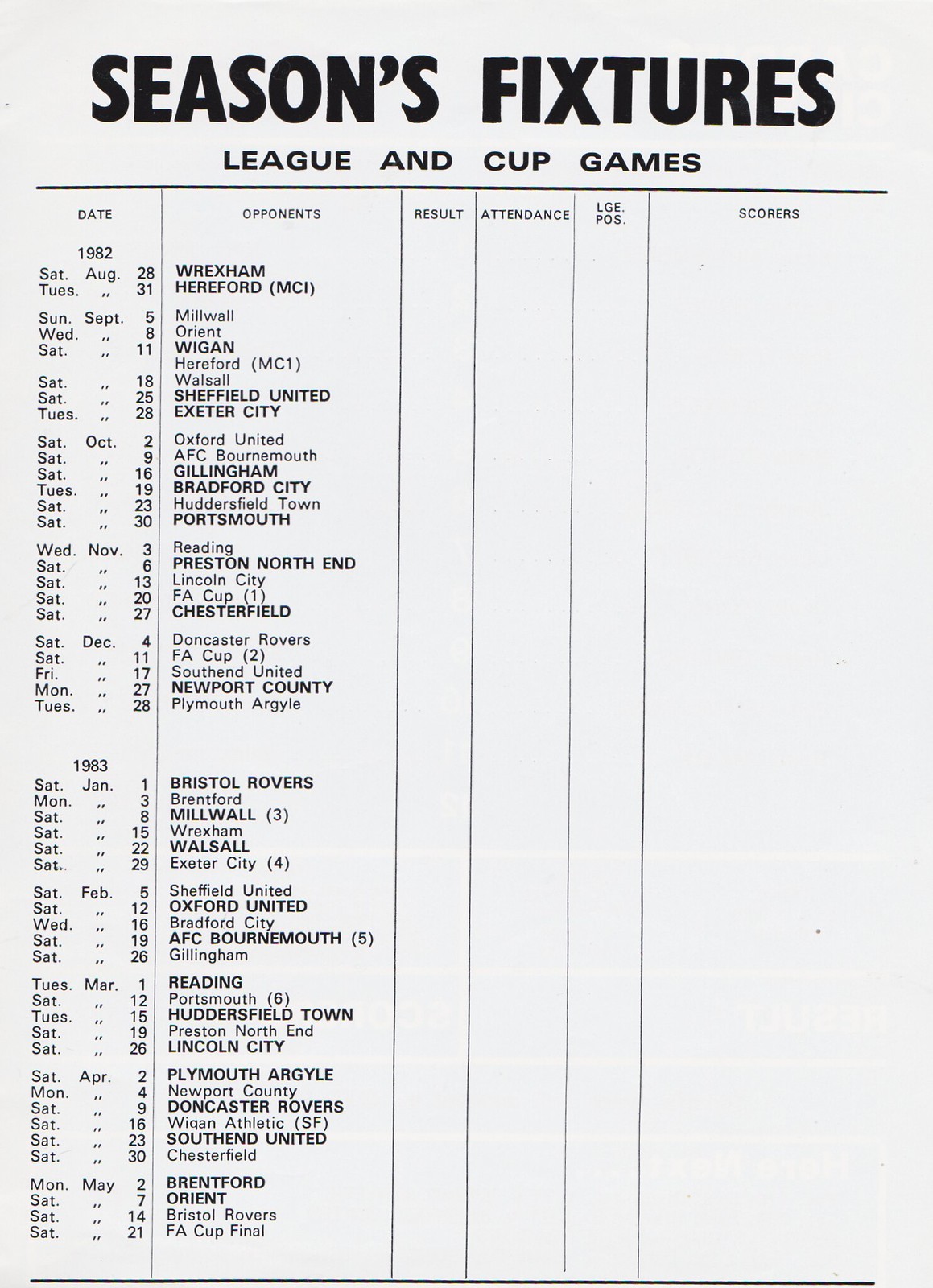The image displays a detailed printout of a season's fixtures in bold, black, capitalized letters at the top, under which it states "League and Cup Games." The table below is divided into six columns with headers labeled Date, Opponents, Result, Attendance, Lge.Pos., and Scorers. The schedule spans from August 28, 1982, to May 21, 1983, with dates for the 1982 part running from Saturday, August 28th to Tuesday, December 28th, and the 1983 segment running from Saturday, January 1st to Saturday, May 21st. Opponents are listed prominently, including teams such as Wrexham and Hartford. The layout resembles a spreadsheet, and while the boxes for Result, Attendance, Lge.Pos., and Scorers are currently empty, they are clearly intended to be filled in. The entire schedule is set against a plain white background, emphasizing the structured, organized appearance of the fixture list.